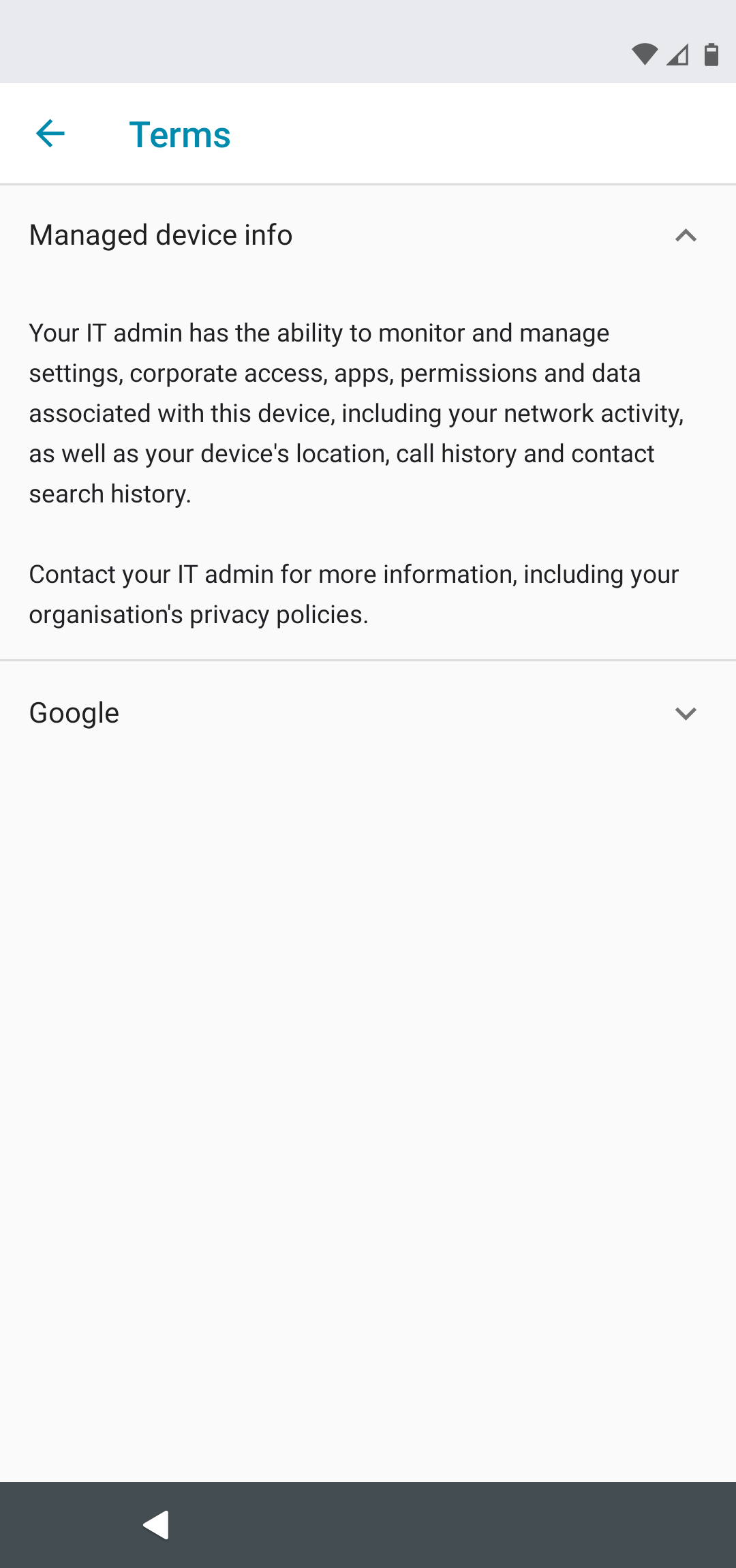This image is a screenshot captured from a cell phone, featuring various UI elements and informational text. At the top of the screenshot, a light gray status bar contains icons in the right-hand corner. The first icon is a dark gray triangle symbol. Next to it is a right-angled triangle with two 45-degree angles, shaded gray at its base. Adjacent to these is a gray battery icon, indicating that the battery is three-fourths full.

Below the status bar is a thin white line, above which "Terms" is written in blue letters, accompanied by a left-pointing arrow. The main portion of the screenshot details a message under the heading "Manage Device Info." The message informs the user that their IT administrator has the capability to monitor and manage various settings, including corporate access, apps, permissions, and data associated with the device. This includes monitoring network activity, device location, call history, and contact search history. Users are advised to contact their IT admin for further information, including organizational privacy policies.

Further down, a section labeled "Google" is marked by a right-pointing arrow. The lower half of the image is predominantly white space, save for a gray bar at the very bottom. This bar has a white left-pointing arrow, suggesting a navigation option.